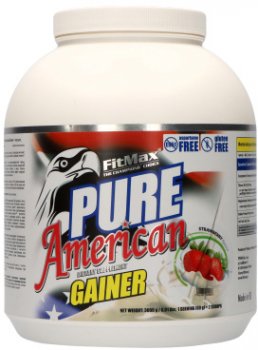This photograph showcases a product against a seamless white background that extends infinitely, eliminating any visible frame or edges. The product in focus is branded as "Pure American"; its label prominently features patriotic imagery, including an eagle, strawberries, red and white stripes, and white stars on a blue background. The product name "Fit Max" is clearly displayed, with "Gainer" written underneath, suggesting it is a dietary supplement. The label also includes text indicating some sort of promotional or quality assurance message, although the specifics are unreadable. The detailed product information runs along both the right and left edges of the label, providing comprehensive details about the supplement.